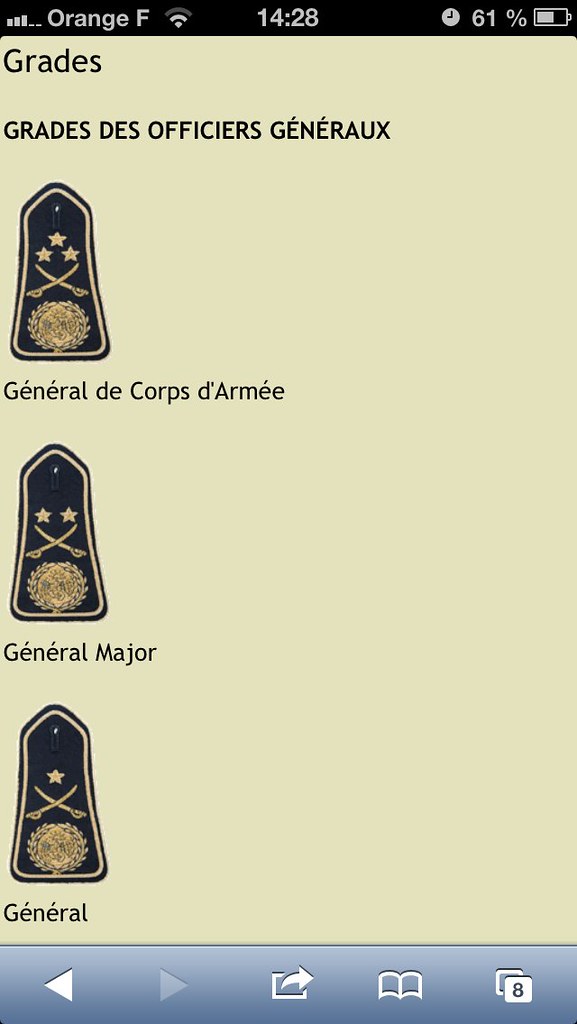The image is a screenshot taken from a phone, displaying military rank insignias in French. The phone status bar at the top shows the local time, signal strength with three orange bars, and the battery level at 61%. The background of the image is off-white or tan. The screenshot showcases three distinguished military grades, each represented by black shield patches with tan details. 

At the top, the text reads "Grades De Officiers Genéraux" in black. The highest rank is highlighted by a patch displaying a globe surrounded by laurels with three stars above, and a pair of crossed sabers at the center, labeled "Général De Corps D'armée." The rank below has a similar design featuring two stars and is labeled "Général De Division." The lowest rank uses the same emblematic shield but has only one star, labeled simply "Général."

At the bottom of the phone screen, hints of a browser interface are visible, including a blue bar, back button, and a button to open multiple pages.